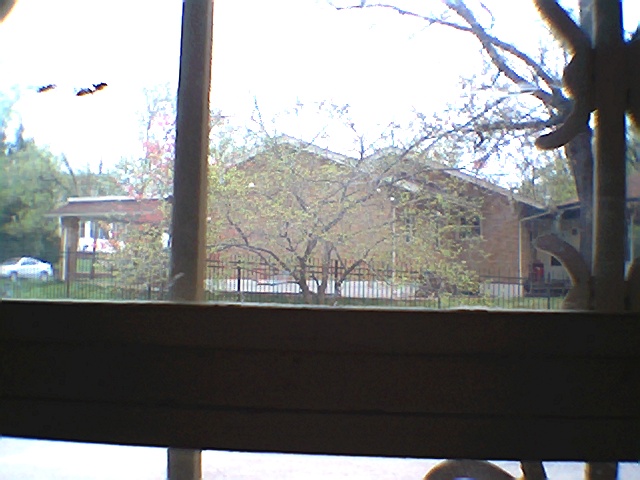This detailed color photograph was taken from inside a house, through a window framed with a black horizontal window pane at the bottom and two vertical wooden bars. Additional curved bars indicate some sort of iron grating. Outside, a gray, hazy sky looms over a grassy area that features an iron bar fence running across it. Beyond the fence lies a parking lot with a single car facing towards the camera. The main focus is a modest brick house with a double gabled roof and an awning on the left side adorned with reddish tiles. A tree with long spreading branches and small leaves, suggesting early spring, stands prominently in front of the house. In the distant background, a white house is also visible. There's ample sunlight indicating the picture was taken during the day, despite the overcast skies.